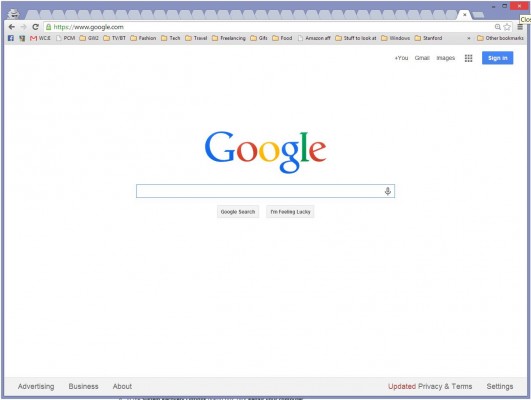The image depicts the main screen of the Google search page. Dominating the top is the iconic Google logo, featuring a capital 'G' in blue, followed by two 'O's — one red and one yellow, a lowercase 'g' in blue, a lowercase 'l' in green, and a lowercase 'e' in red. Below the logo is a rectangular search bar with a microphone icon positioned at its right end. Underneath the search bar, there are two options: "Google Search" and another box that appears to read "I'm Feeling Lucky."

At the top of the page, multiple browser tabs are open, indicating other searches or webpages being accessed. In the upper right-hand corner, there are links labeled "Gmail," "Images," and a grid icon that opens a menu of various Google apps. Next to these links is a blue "Sign in" button. 

Towards the bottom of the screen, the left side displays links to "Advertising," "Business," and "About." On the right side, links are provided for "Privacy," "Terms," and "Settings," detailing Google's policies and options for the user.